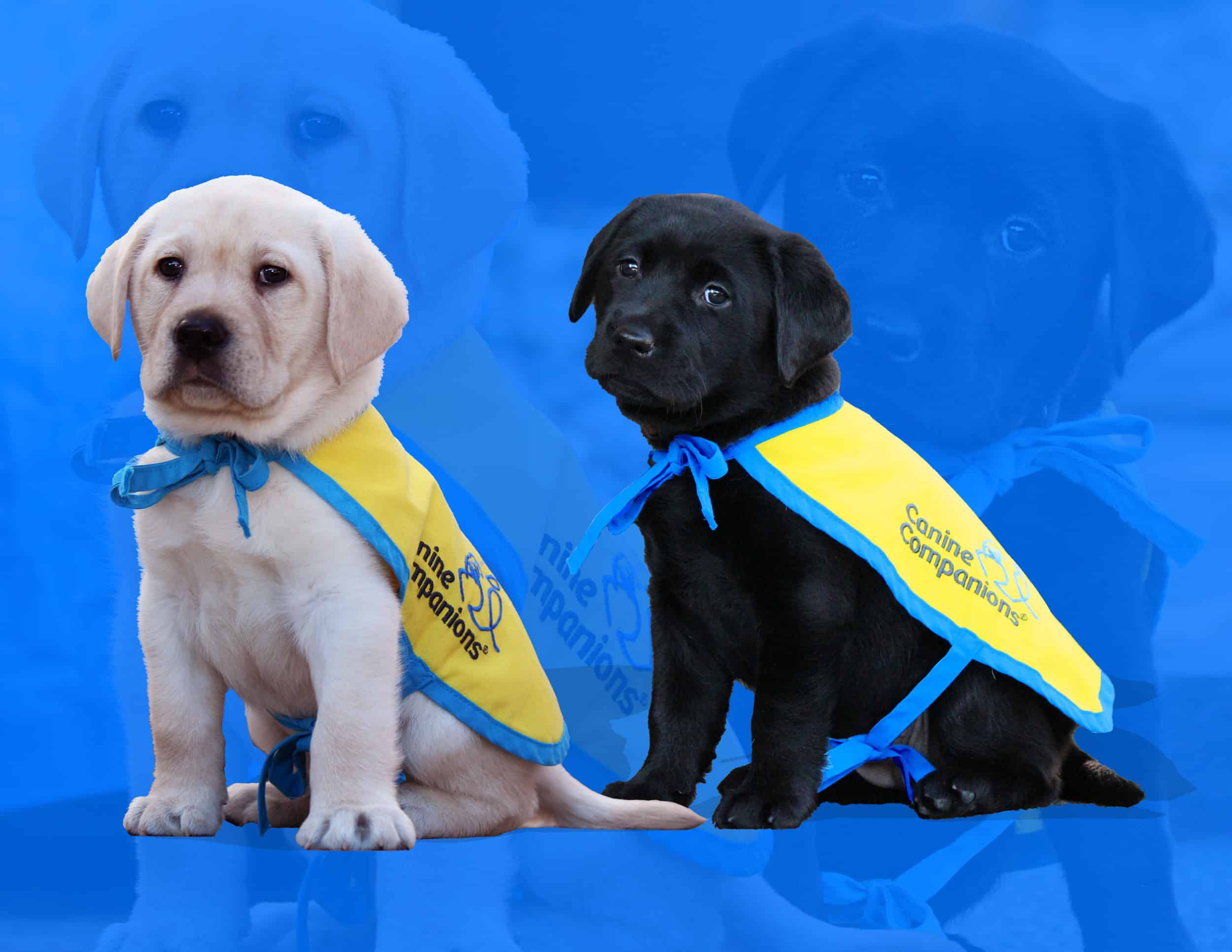In the foreground of this image, two puppies pose adorably. The puppy on the left is white with large paws and droopy cheeks, resembling a young Labrador, and looks directly at the camera. The puppy on the right is black, also resembling a Labrador, and gazes slightly to the side. Both puppies are dressed in yellow capes trimmed with blue, which feature the words "Canine Companions" along with a blue logo, indicating they are being trained for assistance. The background features a significantly dimmed, enlarged, and blue-hued version of the same puppies sitting and looking ahead with somewhat sad expressions. The overall effect creates a heartwarming and poignant scene showcasing the endearing puppies destined for a greater purpose.